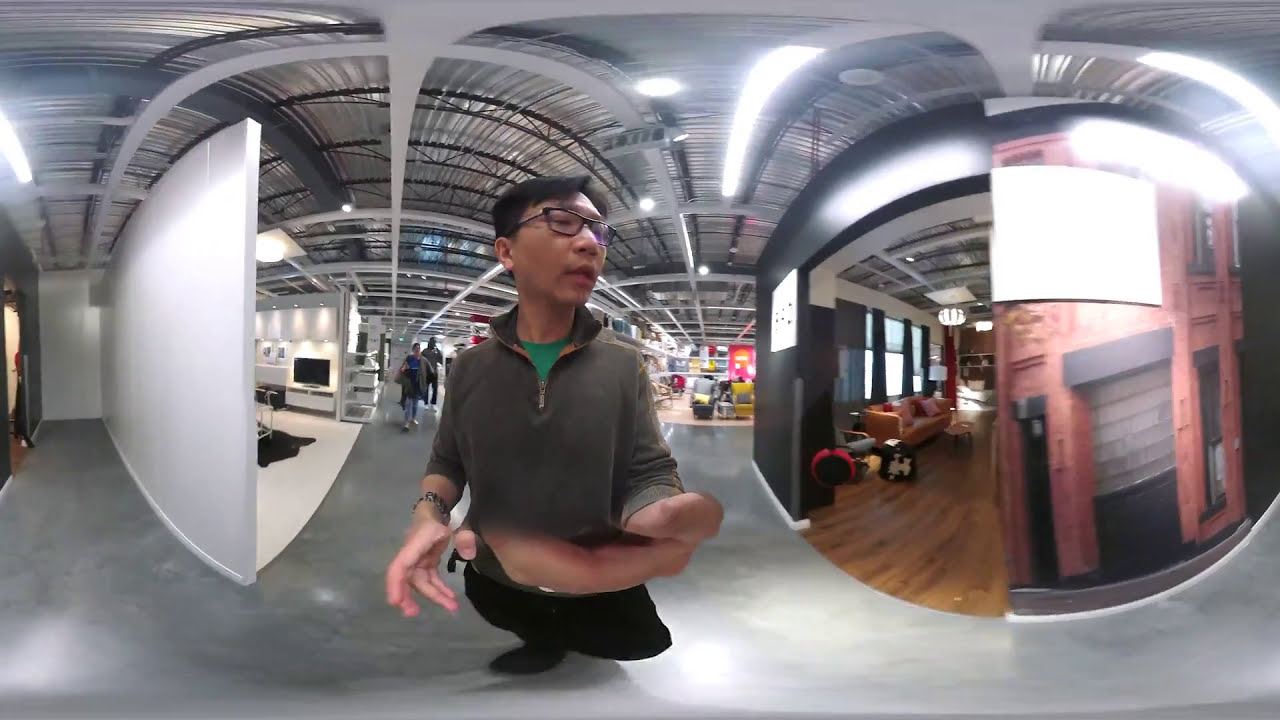The photograph captures a panoramic, slightly distorted image of a man in an industrial setting, possibly a warehouse-like store with a metallic, silver ceiling featuring steel rafters and industrial fluorescent lights. The man, who is Asian with black hair and wearing clear-lens black glasses, is dressed in an olive green quarter-zip sweater over a kelly green t-shirt, black pants, and black shoes. His left arm is outstretched towards the camera, suggesting he might be the one taking the photo, and he appears to be gesturing with his right hand. The floor beneath him is silvery gray, matching the industrial aesthetic. To his right, a room with wooden floors and an orange couch is visible, partially separated from the industrial section. On the left is a white wall that features a black screen and recessed lighting. Behind him, blurred figures of a man and a woman suggest an active environment, possibly a large store or warehouse. Further to the right, a mural of a red brick building against a black wall adds to the setting's eclectic appearance.